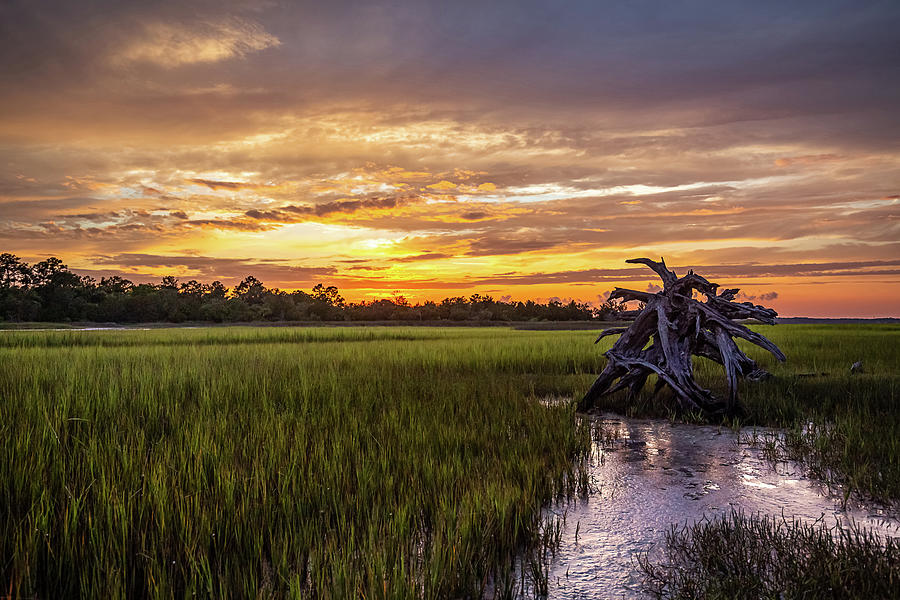A professionally shot outdoor landscape photo captures a picturesque swampland at dusk. In the foreground, tall, vibrant green grasses rise around patches of reflective water, which is scattered throughout the swampy terrain. Dominating the foreground is an aged, contorted tree trunk with a bluish-white and brown hue, resembling a piece of driftwood. This dead tree stands prominently against the serene water backdrop, its bare, gnarled branches adding a dramatic element to the scene. Behind the tree, the flat, expansive field leads to a distant tree line comprised of lush, dark silhouettes of deciduous trees against the sky.

The skyline is a mesmerizing showcase of natural colors at sunset - swirls of gray and purple clouds intermingle with dramatic bursts of orange, red, yellow, pink, and peach, casting a warm, glowing light over the entire landscape. The sunset sky, densely clouded with these vibrant hues, reflects subtly in the water patches, enhancing the scene's serene beauty. The photograph is devoid of any people, animals, or text, focusing purely on the untouched splendor of nature.